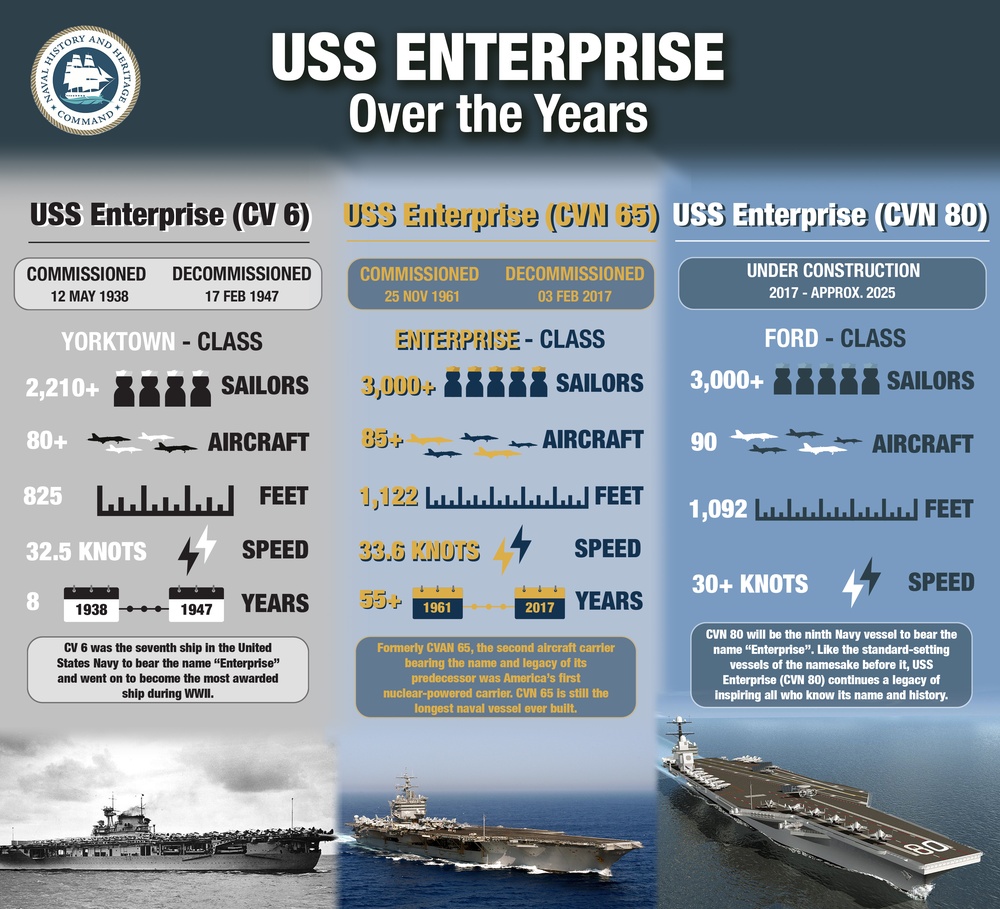The poster, labeled "USS Enterprise Over the Years," includes detailed information and visuals of three iterations of the famous naval vessel, each from different eras. At the top, the title appears in white font against a dark blue background, next to the Naval History and Heritage Command logo in the top left with "Naval History" and "Heritage Command" inscribed within concentric circles. The poster is divided into three distinct sections, each dedicated to a different ship named USS Enterprise.

The first section details the USS Enterprise (CV-6) with a gray background. It specifies that this Yorktown-class aircraft carrier was commissioned on May 12, 1938, and decommissioned on February 17, 1947. It held 2,210 sailors, carried over 80 aircraft, measured 825 feet, and reached speeds of 32.5 knots. Notably, this was the seventh ship in the U.S. Navy to bear the name Enterprise and earned distinction as the most awarded ship of World War II. A black-and-white photograph of CV-6 on the water is showcased at the bottom of this section.

The middle section, under a light blue background, describes the USS Enterprise (CVN-65). This Enterprise-class carrier was commissioned on November 25, 1961, and decommissioned on February 3, 2017. It supported 3,000 sailors, housed 85 aircraft, spanned 1,122 feet, and achieved speeds of 33.6 knots. CVN-65 was the first nuclear-powered aircraft carrier and is still the longest naval vessel ever built. A vivid image captures CVN-65 under a light blue sky with a dark blue sea backdrop.

The final section on a dark blue background covers the USS Enterprise (CVN-80), which is currently under construction from 2017 with an estimated completion around 2025. This Ford-class carrier will accommodate 3,000 sailors, 90 aircraft, span 1,092 feet, and exceed speeds of 30 knots. It will be the ninth naval ship to carry the Enterprise name. At the bottom, a picture portrays the anticipated appearance of CVN-80 on murky greenish-blue waters.

Each section includes the ship’s specifications such as crew capacity, aircraft capacity, dimensions, speed, and historical notes, with photos of the ships providing a visual context at the bottom.